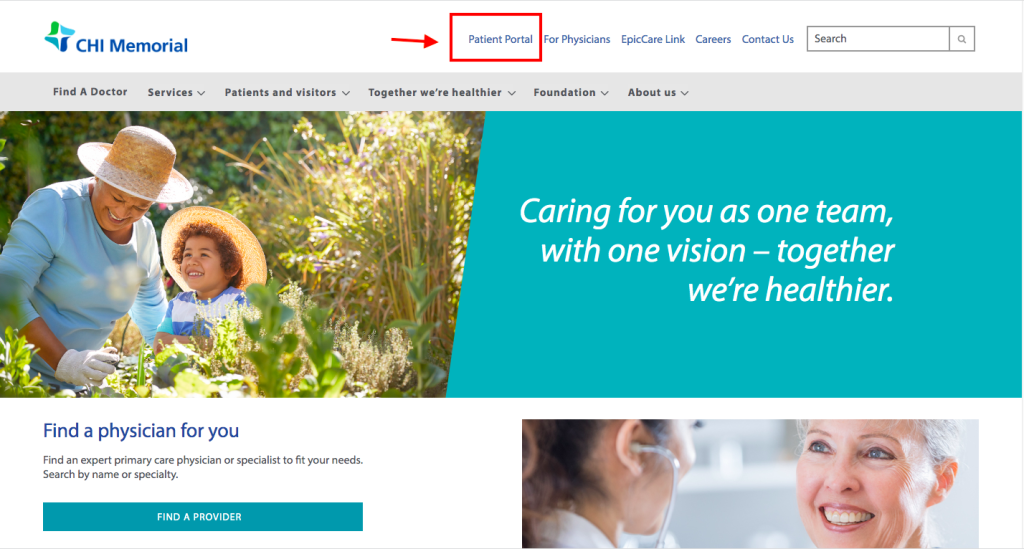The screenshot captures the homepage of the CHI Memorial website. In the top left corner, the CHI Memorial logo is prominently displayed. The header row features several text links: Patients Portal, highlighted with a red box and a red arrow pointing to it, followed by links to Four Physicians, Epic Care Link, Careers, and Contact Us. On the top right side of the same row is a search box.

Below this header is a secondary navigation row with additional links: Find a Doctor, Services (with a dropdown menu), Patients and Visitors (with a dropdown menu), Together We're Healthier (with a dropdown menu), Foundation (with a dropdown menu), and About Us (with a dropdown menu).

The main section of the page features a split hero image. On the left side, an older woman and a young child are joyfully planting plants in a garden. On the right side, the background is teal with the text "Caring for You as One Team with One Vision. Together We're Healthier."

Further down, another row is divided into two sections. The left side contains text encouraging visitors to "Find a Physician for You. Find an expert primary care physician or specialist to fit your needs. Search by name or specialty," accompanied by a "Find a Provider" button. The right side displays the upper half of an image featuring a female doctor with a stethoscope in her ears and an older woman smiling at her.